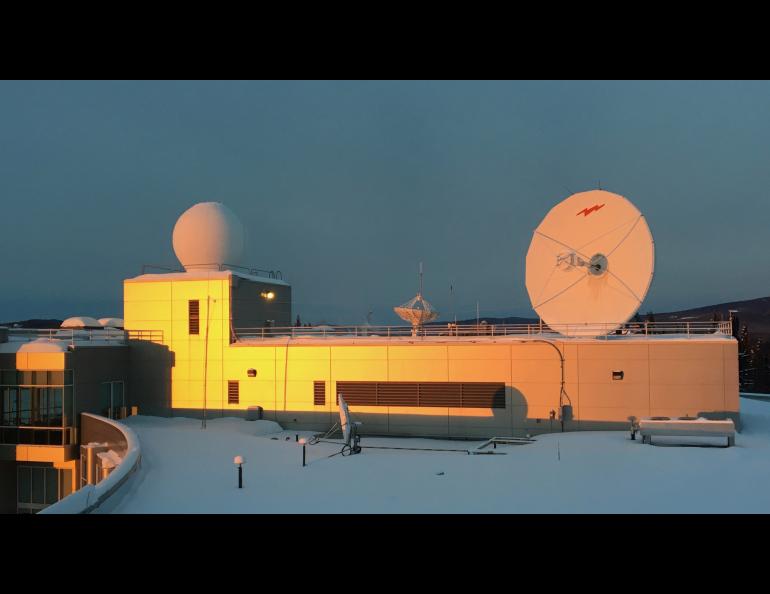The photograph captures a technologically sophisticated facility situated atop a large, colorfully painted building that houses multiple satellite dishes and antennas. Predominantly featuring hues of green and pink that shift to yellow and dark pink in various lighting, the building's structure includes a prominent balcony where a smaller dish and outdoor lighting can be seen. The entire scene suggests a rooftop view, framed by wide vertical black stripes at both the top and bottom of the image. To the right side of the image, a large satellite dish is directed towards the opposite side, while another dish in the center is angled upward into the sky. A dome-like spherical structure, possibly a Doppler radar, is perched on the left side of the building. The roof appears white, likely blanketed in snow, further accentuated by the dark blue, almost grayish, sky indicative of either early morning or late evening light. The photograph impeccably combines architectural and technological elements against the backdrop of a cold, wintry sky.